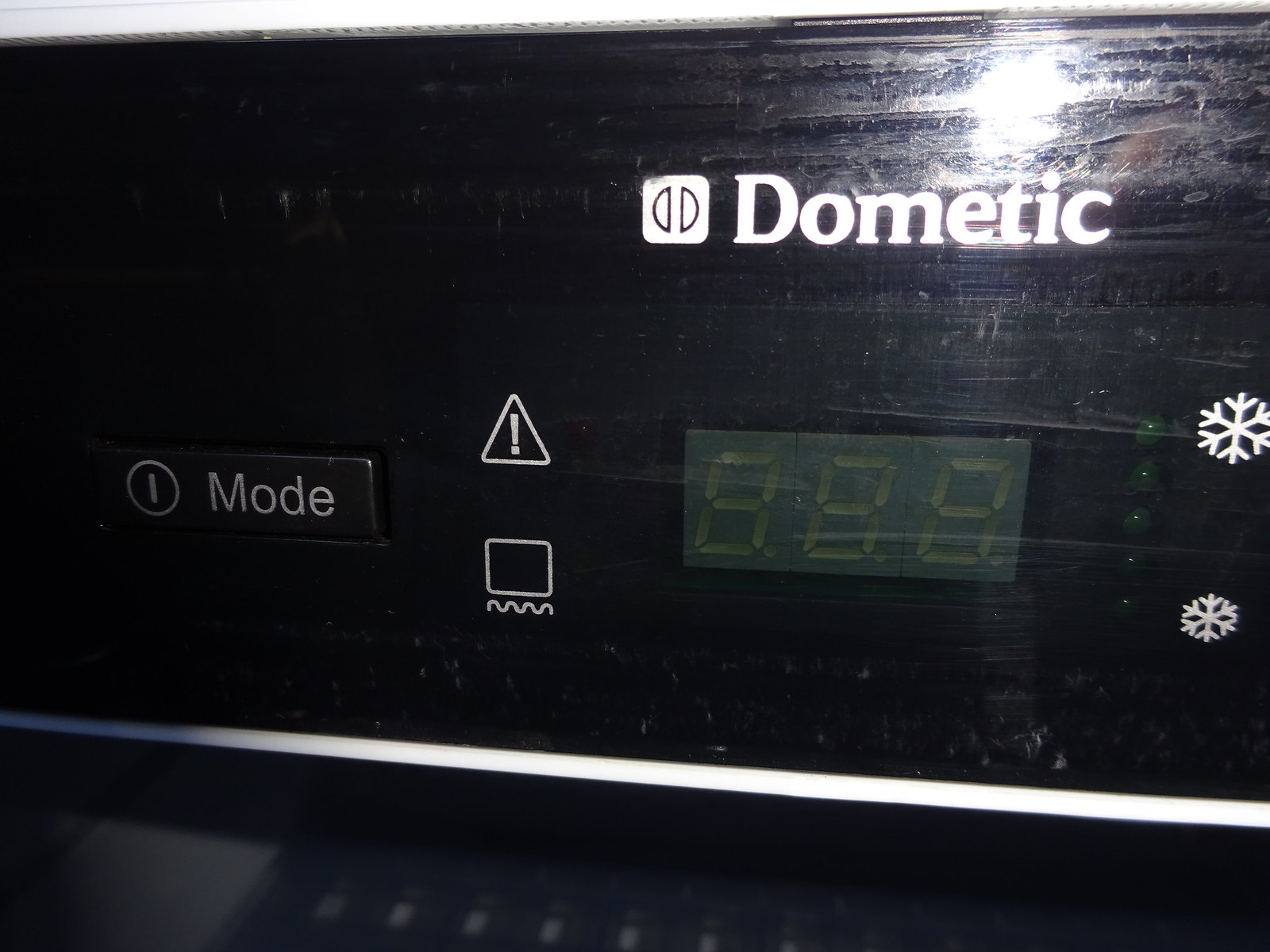This photograph captures an extreme close-up of the front display panel of an electronic device, possibly an air conditioner or a VCR. The display panel, crafted from flat black plastic, features several white pictograms, including an exclamation point inside a triangle and a square on top of a wavy line. Additionally, there are snowflake icons — a larger one at the top and a smaller one at the bottom — accompanied by five vertical green lights, likely indicating the cooling level. The panel also sports an unlit LED display that currently reads '888' and appears similar to an alarm clock display. The upper part of the panel has the word 'Dometic' printed in white, perhaps indicating a non-English-speaking manufacturer's attempt to mimic the word 'domestic.' To the left, a button labeled 'mode' is visible.